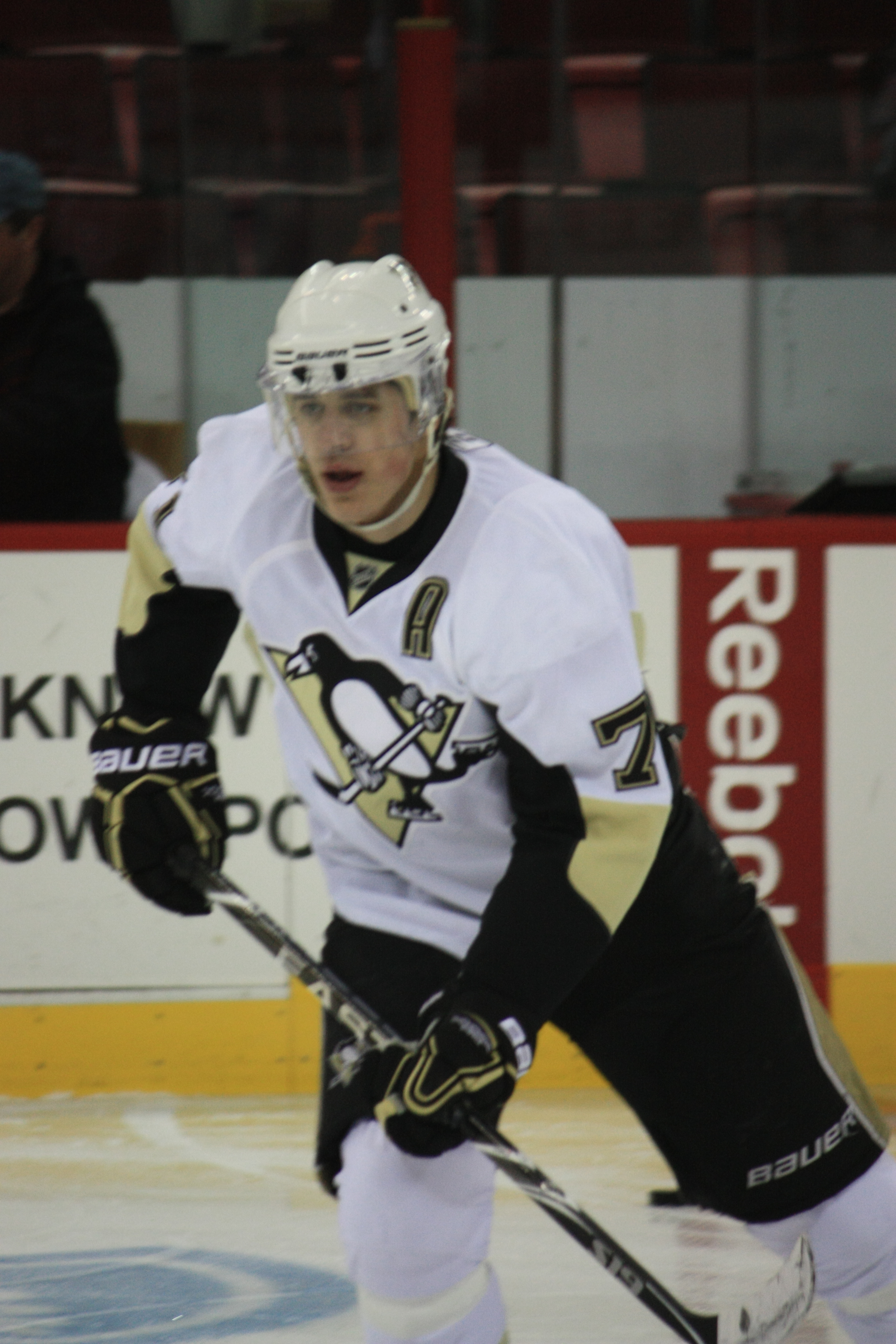This detailed photograph captures a white-helmeted ice hockey player in mid-motion, skating towards the viewer and slightly to the left on an ice rink. The player is donning a white jersey featuring the Pittsburgh Penguins logo on the chest, coupled with black pants that are white at the bottoms, black gloves with gold detailing, and the word "Bauer" inscribed in white letters. He is firmly grasping a hockey stick, with his right hand holding the top and his left hand gripping closer to the bottom. His black shorts are worn over white leggings, and the helmet showcases a clear face shield secured by a white strap under his neck. The background reveals the rink's wall, which is yellow at the base and white above, adorned with various advertisements, including a noticeable red "Reebok" text to the player's right. Beyond the wall, there's a series of glass panes, and in the stands, which appear mostly empty, a solitary figure is partially visible to the left. An emblem can be seen in the left bottom corner of the icy surface beneath the player.